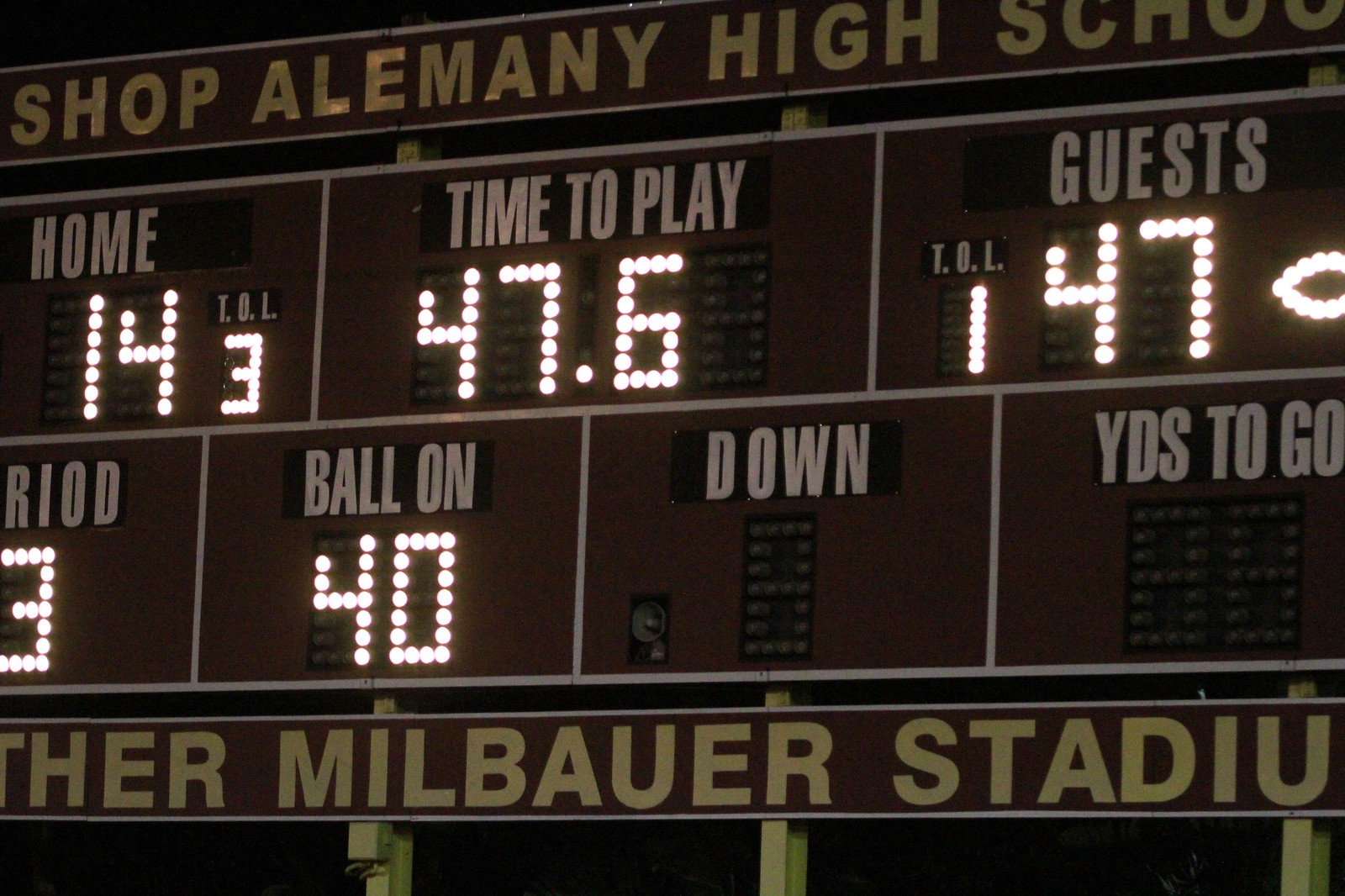This photograph captures a close-up view of a dark-colored electronic scoreboard at a football game, presumably at Milbauer Stadium. The top of the scoreboard prominently displays bold, capitalized text reading "SHOP ALEMANEY HIGH SCHOOL." The board's illuminated numbers reveal the game's details: on the left, it shows "HOME" with a score of 14 and "T.O.L" (presumably time-outs left) indicating 3. The center of the scoreboard highlights "TIME TO PLAY" with 47.6 seconds remaining. On the right side, "GUESTS" have a score of 47 and "T.O.L" marked as 1. Below this, it indicates "PERIOD 3" and "BALL ON 40," suggesting the game's current progress. Notably, there are fields for "DOWN" and "YARDS TO GO" which are currently not illuminated or showing any numbers. The bottom portion of the scoreboard, though partially obscured, appears to read "MILBAUER STADIUM." The numbers and texts are displayed in little dot lights, and the descriptive letters at the top and bottom are in a faded gold color.